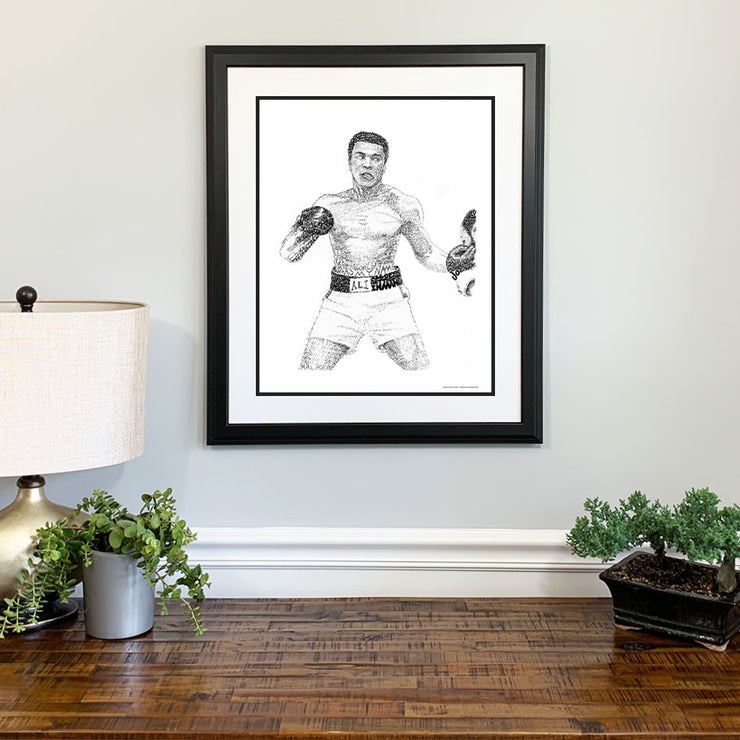This interior photo features a framed pencil sketch of Muhammad Ali in a fighting pose, prominently displayed on a light gray wall with white trim. The detailed artwork shows Ali from the thighs up, standing in a wide stance, donned in boxing shorts labeled "Ali," and preparing to throw a punch at an unseen opponent. The drawing is framed with a white mat and a sleek black border and includes some type of lettering in the bottom right corner. The table below the artwork is made of wood and holds a small bonsai tree in a black pot to the right, and a fern or green foliage in a silver cylindrical pot closer to the center. To the left of the plants, a lamp with a circular golden base, bronze top, and white shade adds a warm glow to the setup.